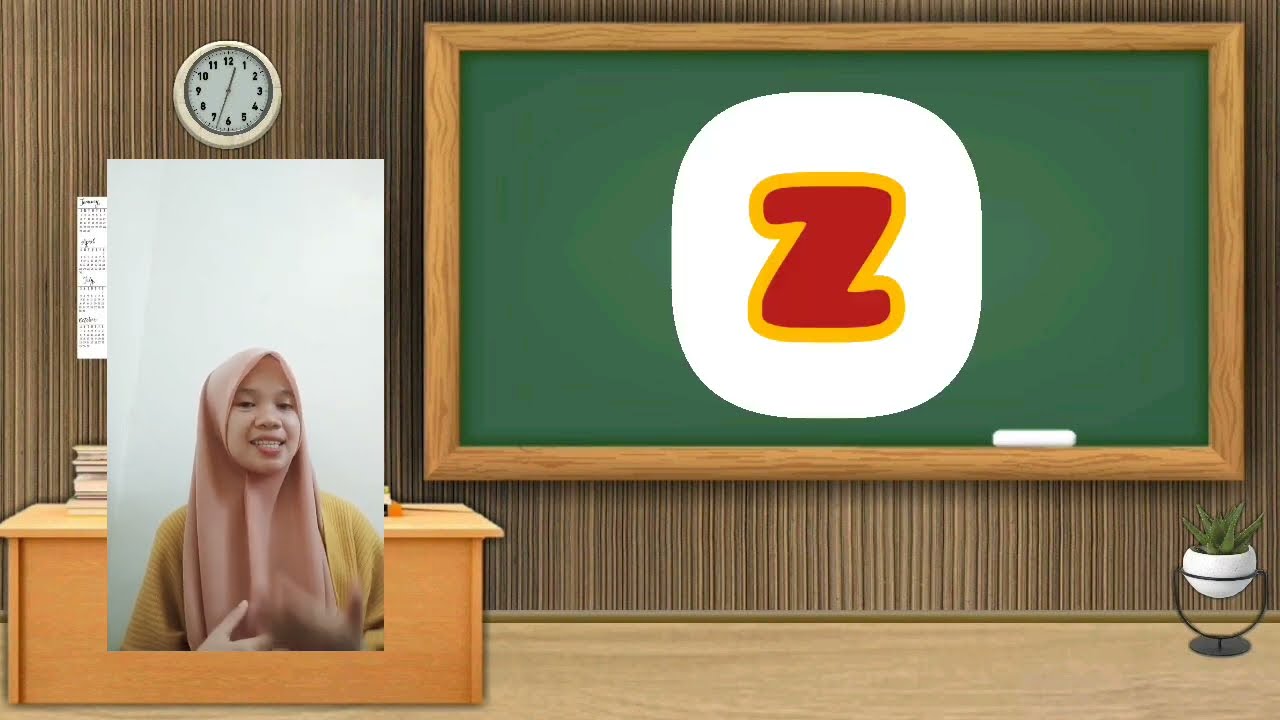The image is a detailed, horizontally aligned, digitally created classroom scene. The background features a wall with narrow vertical wooden strips, highlighting a very large green chalkboard with a thick brown wood border. A piece of white chalk rests on this border. Dominating the chalkboard is a large, circular, white-colored shape with a bold, red 'Z' outlined in yellow. In the upper left corner of the wall, there's a round clock with a white border. Adjacent to the chalkboard on the left, a wooden desk with a stack of papers is visible. Above this desk, there's a photo inset of a light-skinned woman, possibly of Asian origin, wearing a light pink hijab and a yellow sweater. Her mouth is open in a smile, suggesting she might be speaking. Below and to the right of the desk, a small aloe vera plant in a white pot sits on a black stand. This scene evokes the setting of an educational presentation or classroom.